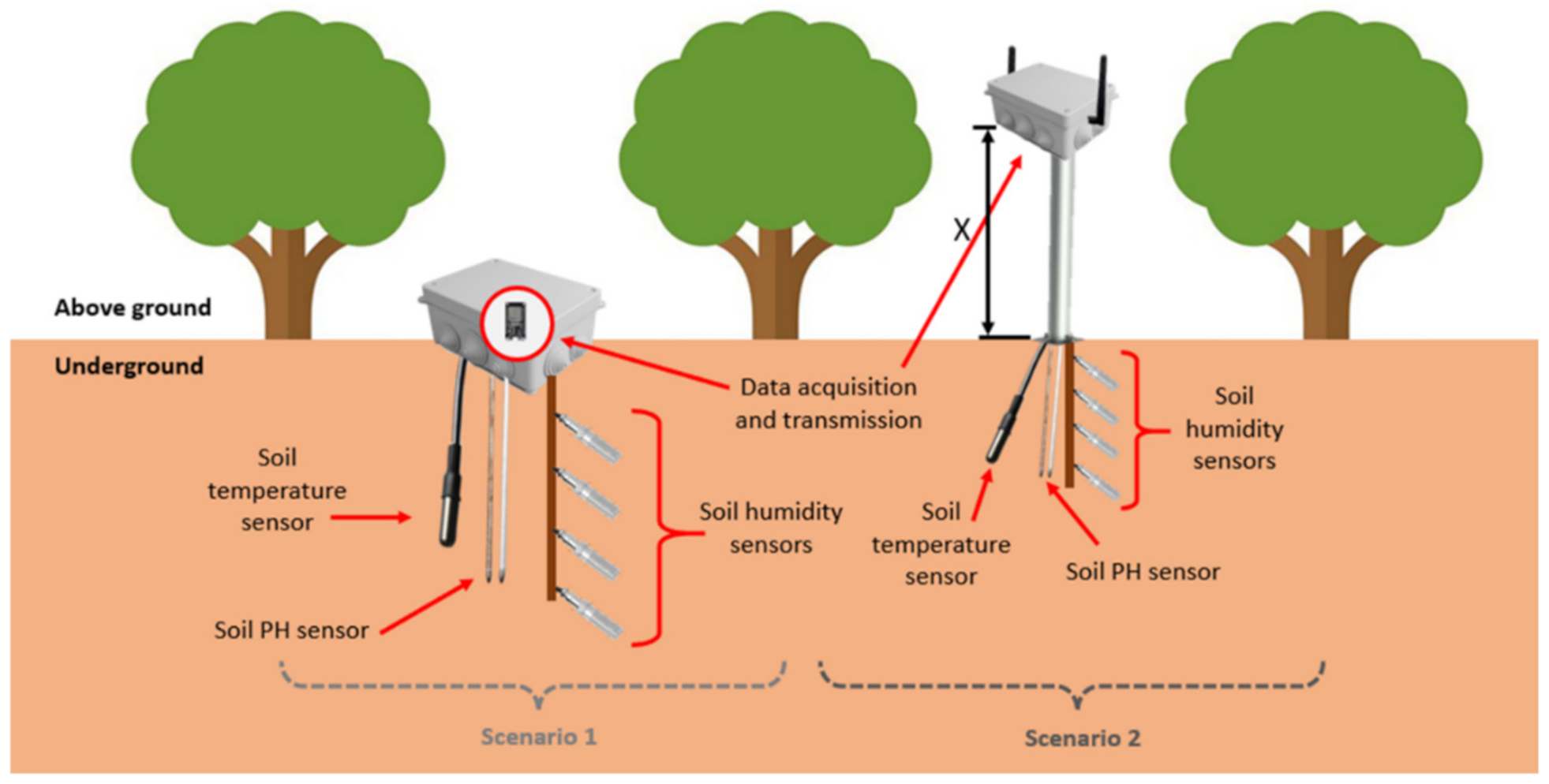The image is an artistically illustrated diagram showing soil testing equipment in a split scene with a white top half labeled "above ground" and a tan bottom half labeled "underground." At the top boundary of the tan area, there are three identical green trees with brown trunks, drawn in a simplistic, child-like style with no leaves. 

On the tan "underground" section, there are various labels and components. A red arrow points to a "soil temperature sensor" embedded in the soil, while a "soil pH sensor" is slightly visible above the surface. Both sensors are connected to a device labeled "data acquisition and transmission." Additionally, "soil humidity sensors" are mounted along a brown stick or tube inserted into the ground. 

On the right hand side, another device labeled similarly is depicted, with a "sensor Wi-Fi apparatus" mounted on an elevated post reaching the height of the trees' tops. The diagram is divided into two scenarios: "scenario 1" with the setup largely underground, and "scenario 2" with an above-ground apparatus. This detailed setup likely illustrates an agricultural application for monitoring soil conditions to ensure optimal tree growth.